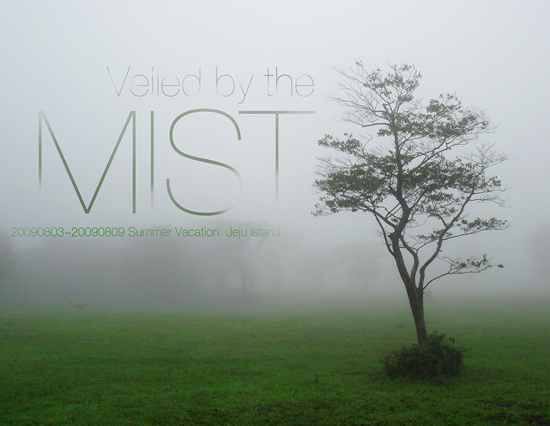The advertisement showcases a serene, mist-filled landscape, capturing a solitary, partially-grown tree standing in a lush expanse of green grass. The prominent tree, not very tall and with sparse branches, is enveloped in a dense layer of fog, shrouding the surrounding area and creating an ethereal atmosphere. The text "Veiled by the Mist" is elegantly overlaid on the mist, adding to the poetic feel of the image. Below this, essential details are inscribed, including "Summer Vacation," followed by "Jeju Island" and what appears to be a date range, "2009.08.03 - 2009.08.09." There are no people or additional landmarks visible, emphasizing the tranquil, untouched beauty of the scenery. This advertisement evokes a sense of peaceful escape, ideal for promoting a summer retreat to Jeju Island.